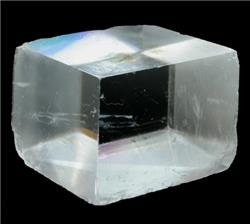This photograph captures a cube-shaped crystal with polished faces set against a completely black background. The crystal, resembling a mineral specimen, features a black square at its center, visible through its transparent sections. Light reflections on the top left of the cube create hints of blue and white hues, while the lower section near the black square shows touches of brown and pink. The cube's surface displays a mix of white, gray, and brown tones due to various scratches and inclusions. Despite its primarily smooth and precise facets, some edges appear rough and irregularly shaped. One of the cube's 90-degree corners faces the viewer, highlighting the intricate structure of this captivating crystalline form. The entire image is framed by a thin black outline.